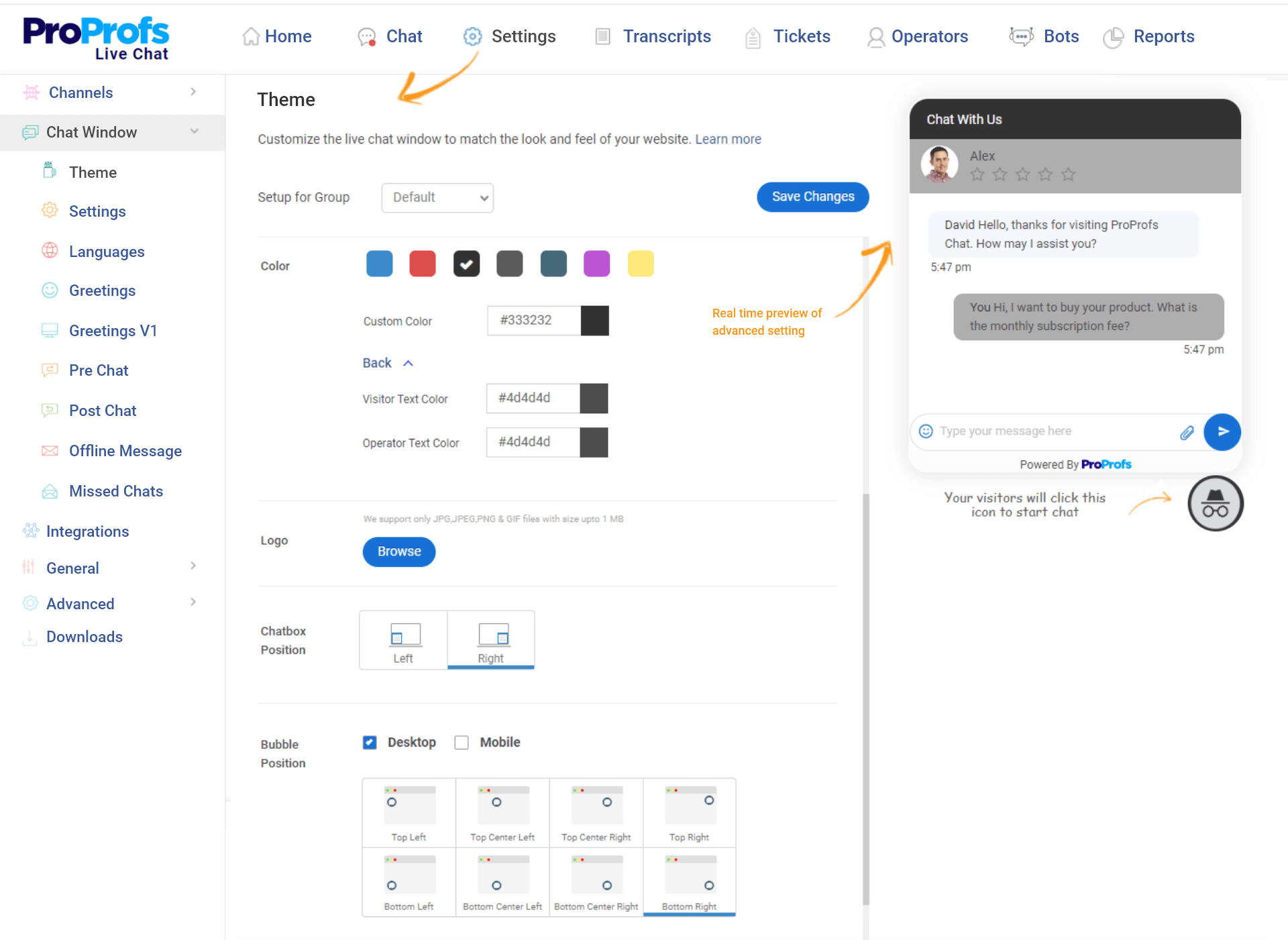A cropped screenshot of the ProProfs live chat feature on a webpage, showcasing an instructional guide. The background is predominantly white. In the upper left corner, the ProProfs logo is prominently displayed, with the words "Live Chat" centered beneath it in small blue font. Adjacent to this, a horizontal navigation menu includes options such as Home, Chat, Settings, Transcripts, Tickets, Operators, Bots, and Reports. The 'Settings' option is emphasized with an orange arrow, directing the viewer's attention.

On the left side of the screenshot, a vertical panel displays various settings categories. The 'Chat Window' category is selected, revealing its subcategory 'Theme', which is accompanied by another orange arrow for emphasis.

To the right, a pop-up chat box features an operator's profile picture, name, and star rating. The chat bubble reads, "Hello, thanks for visiting ProProfs Chat. How may I assist you?" Below, there is a user reply.

Additionally, an annotation on the left of the chat box includes a pointing arrow and the text "Real-time preview of advanced setting," providing further context.

This screenshot serves as an informational guide on navigating and utilizing the settings within the ProProfs live chat feature.